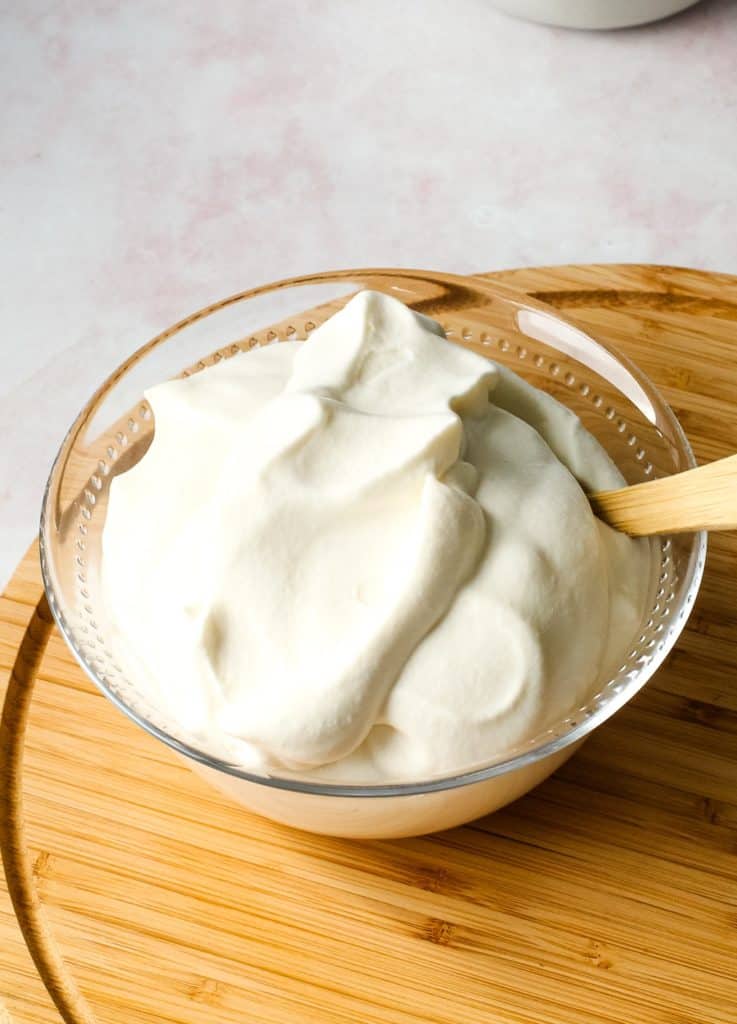The image is a detailed, vertical, rectangular photograph of a glass bowl containing a dense, white, fluffy substance – potentially whipped cream, vanilla yogurt, pudding, or even mayonnaise – that has a thick, textured surface with raised clumps. The bowl features a decorative, curved rim and is situated on the upper left quadrant of a circular wooden tabletop or cutting board, which itself has a groove cut around its edge. The tabletop displays a bamboo-like texture reminiscent of a lazy Susan or serving platter. A wooden spoon is placed in the bowl, its handle slightly visible, suggesting it might be used to scoop the substance. The surface beneath the table is grey and slightly out of focus, balancing the composition of the image.